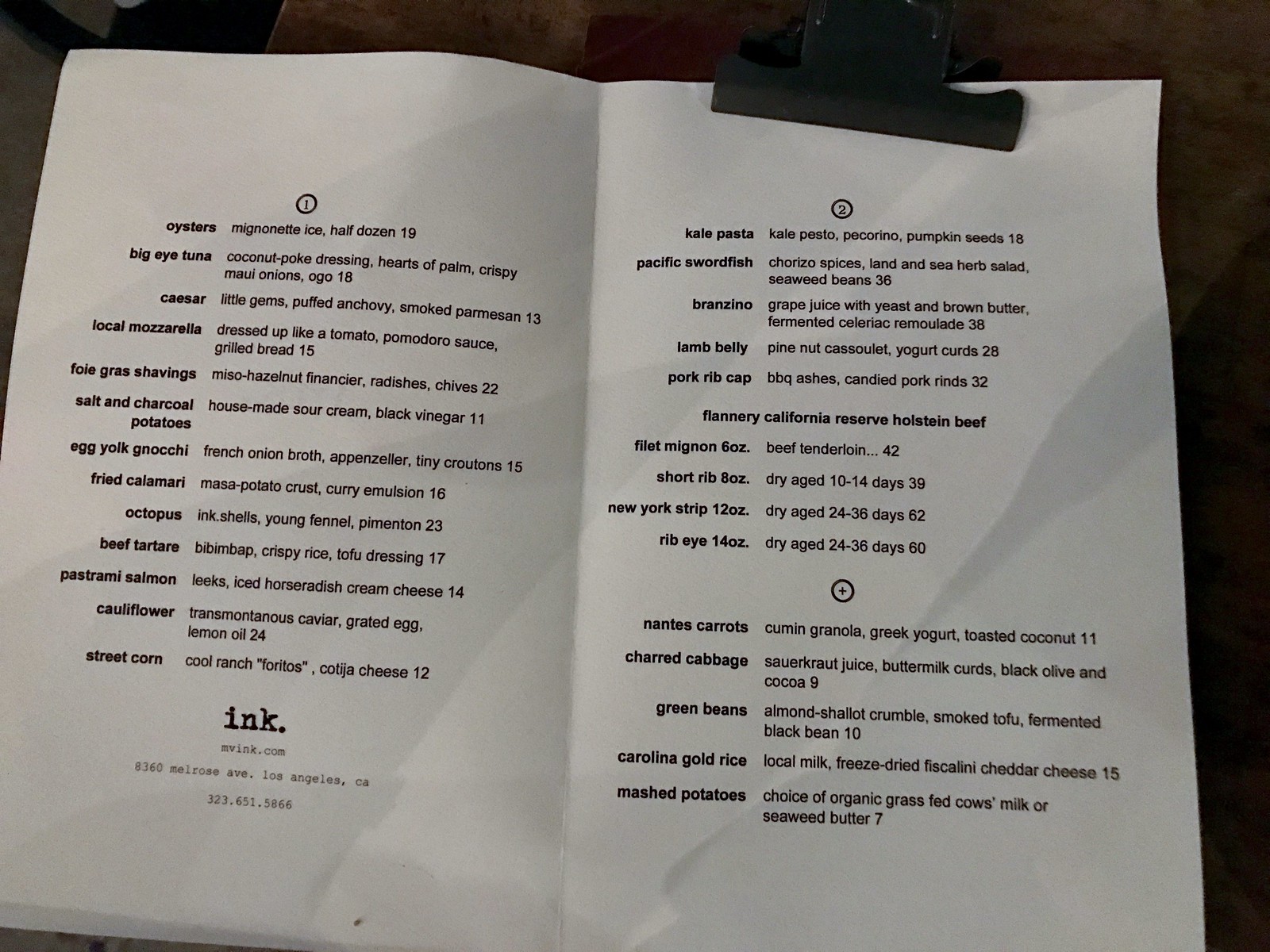The image features a folded white menu secured to a black background with a black bulldog clip. The menu is printed in black ink and is tilted slightly upward to the left. At the bottom of the menu, in lowercase letters, are the words "ink." followed by "nvinc.com", along with the address "8360 Melrose Avenue, Los Angeles, California" and the phone number "323-651-5866."

The left page of the menu, marked with a circled number one, lists the following items: oysters, big eye tuna, Caesar, local mozzarella, foie gras shavings, salt and charcoal potatoes, egg yolk gnocchi, fried calamari, octopus, beef tartare, pastrami salmon, cauliflower, and street corn.

The right page, marked with a circled number two, offers dishes such as kale pasta, Pacific swordfish, branzino, lamb belly, pork rib cap, Flannery's California Reserve Holstein beef, filet mignon (6 ounces), short rib (8 ounces), New York strip (12 ounces), and ribeye (14 ounces). The selection of sides includes Nanta's carrots, charred cabbage, green beans, Carolina gold rice, and mashed potatoes.